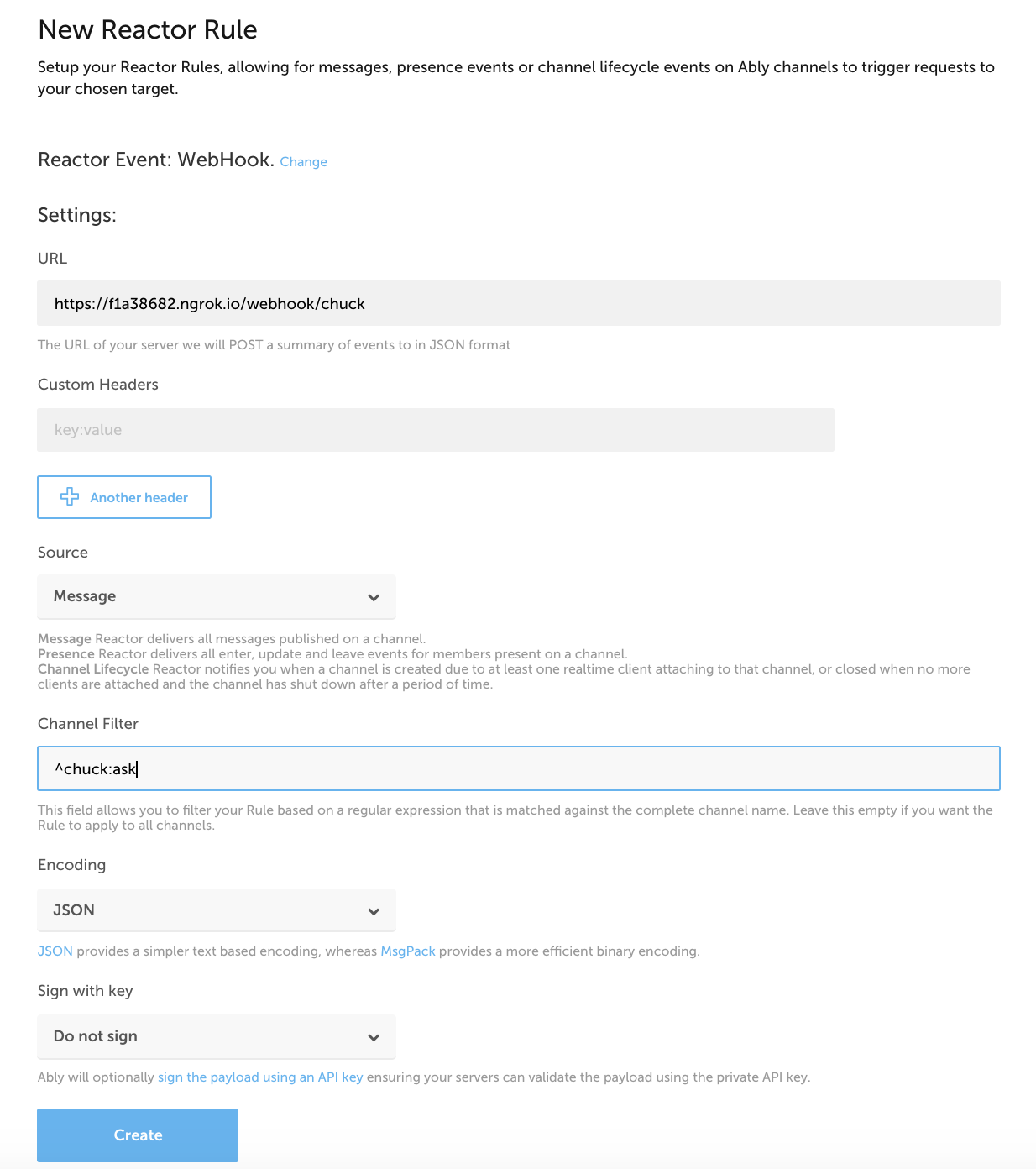**Detailed Caption for Website Screenshot:**

The image showcases a screenshot of a website interface designed for setting up reactor rules in Ably channels. The background of the interface is white, with text predominantly in dark gray and black for visibility. At the top of the interface, there's a prominent heading in bold that reads, "New Reactor Rule."

Below the heading, an explanatory text outlines the purpose of the setup: "Set up your reactor rules, allowing for messages, presence events, or channel lifecycle events on Ably channels to trigger requests to your chosen target."

A subheading titled "Reactor Event Webhook" follows, accompanied by a blue hyperlink labeled "Change."

Another subheading, "Settings," is displayed next. Under this section, a URL field is shown, featuring a light gray box with black text that reads, "https://f1a38682.ngrok.io/webhook/Chuck." Beneath the URL, there's a note in gray text stating, "The URL of your server we will post a summary of events to in JSON format."

The "Custom Headers" section includes a gray box intended for key-value pairs, currently empty with placeholder text indicating "key" and "value." Adjacent to this box is a blue rectangle with a blue plus icon and the text "Add another header."

The next section labeled "Source" contains a drop-down menu set to "Message," and a detailed explanation follows:
- **Message:** "Reactor delivers all messages published on a channel."
- **Presence:** "Reactor delivers all enter, update, and leave events for members present on a channel."
- **Channel Lifecycle:** "Reactor notifies you when a channel is created due to at least one real-time client attaching to that channel or closed when no more clients are attached and the channel has shut down after a period of time."

The "Channel Filter" section includes an input field with a caret indicating a dropdown, currently set to "Chuck: ask." Below this, in gray text, it explains, "This field allows you to filter your rule based on a regular expression that is matched against the complete channel name. Leave this empty if you want the rule to apply to all channels."

Next, "Encoding" is listed with a drop-down menu set to "JSON." An informational text beneath this states, "JSON provides a simpler text-based encoding, whereas MsgPack provides a more efficient binary encoding."

Another section, "Sign with Key," includes a drop-down menu currently set to "Do not sign." The accompanying note explains, "Ably will optionally sign the payload using an API key, ensuring your servers can validate the payload using the private API key."

At the bottom of the interface, there is a blue-turquoise box with white text that says, "Create."